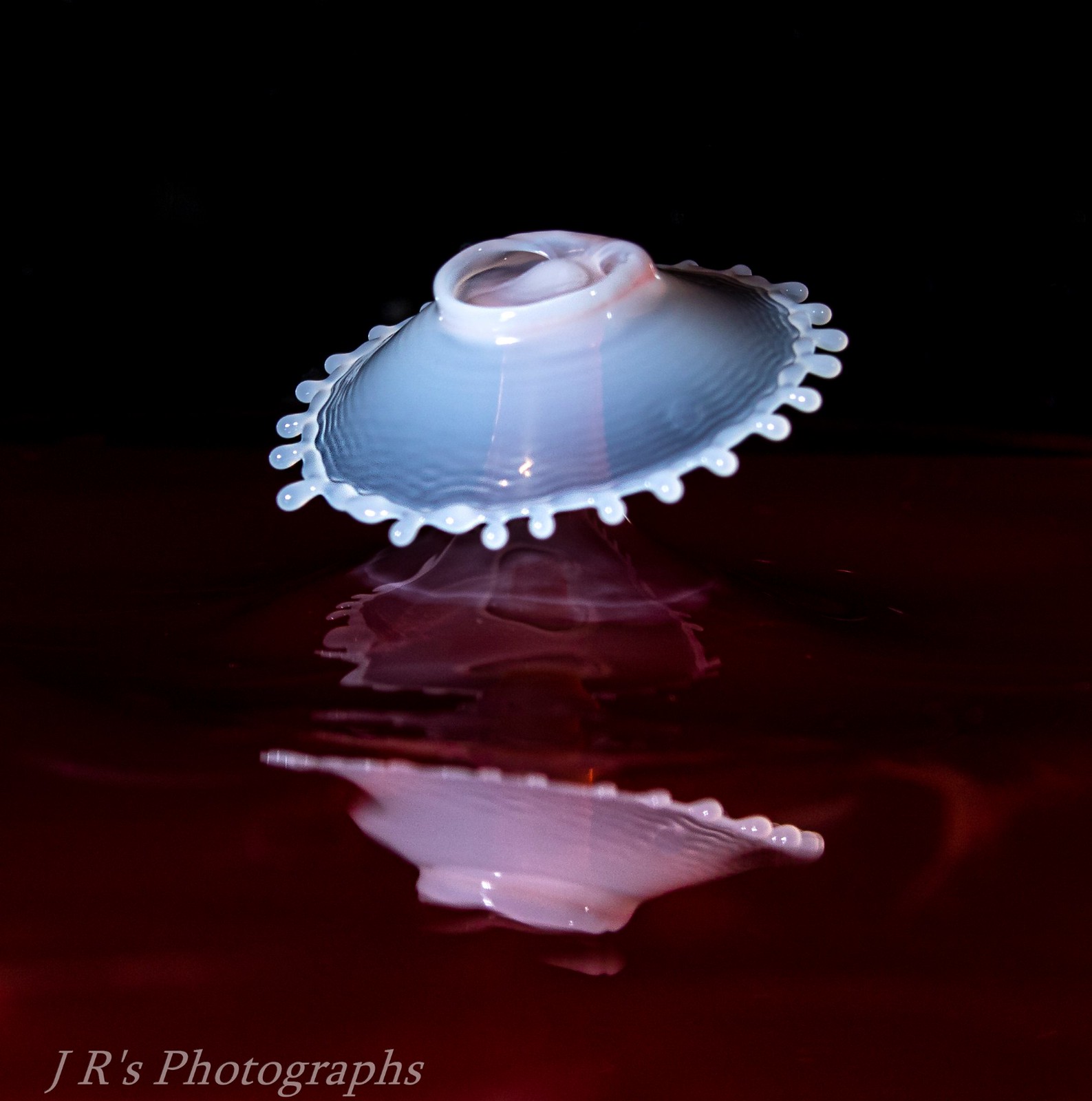The photograph features an intricately designed white object as its focal point, which appears to be either suspended in mid-air or just touching the surface below. The object has a detailed, ridged structure that resembles a conical shape, possibly akin to a volcano or a climbing fountain, and it has an opening at the top, reminiscent of a crown. Surrounding the object's base, the structure descends in slopes and gradually transitions from white to blue, forming ripple-like features around the edges. The object is adorned with numerous droplets, resembling water or raindrops, flying out from its sides, giving an impression of dynamic motion. Reflecting below this centerpiece, the surface captures these elements and is tinged with dark red or maroon hues, likely influenced by the surrounding lighting. The name "J.R.'s Photographies" is inscribed in the bottom right corner, identifying the photographer or studio.